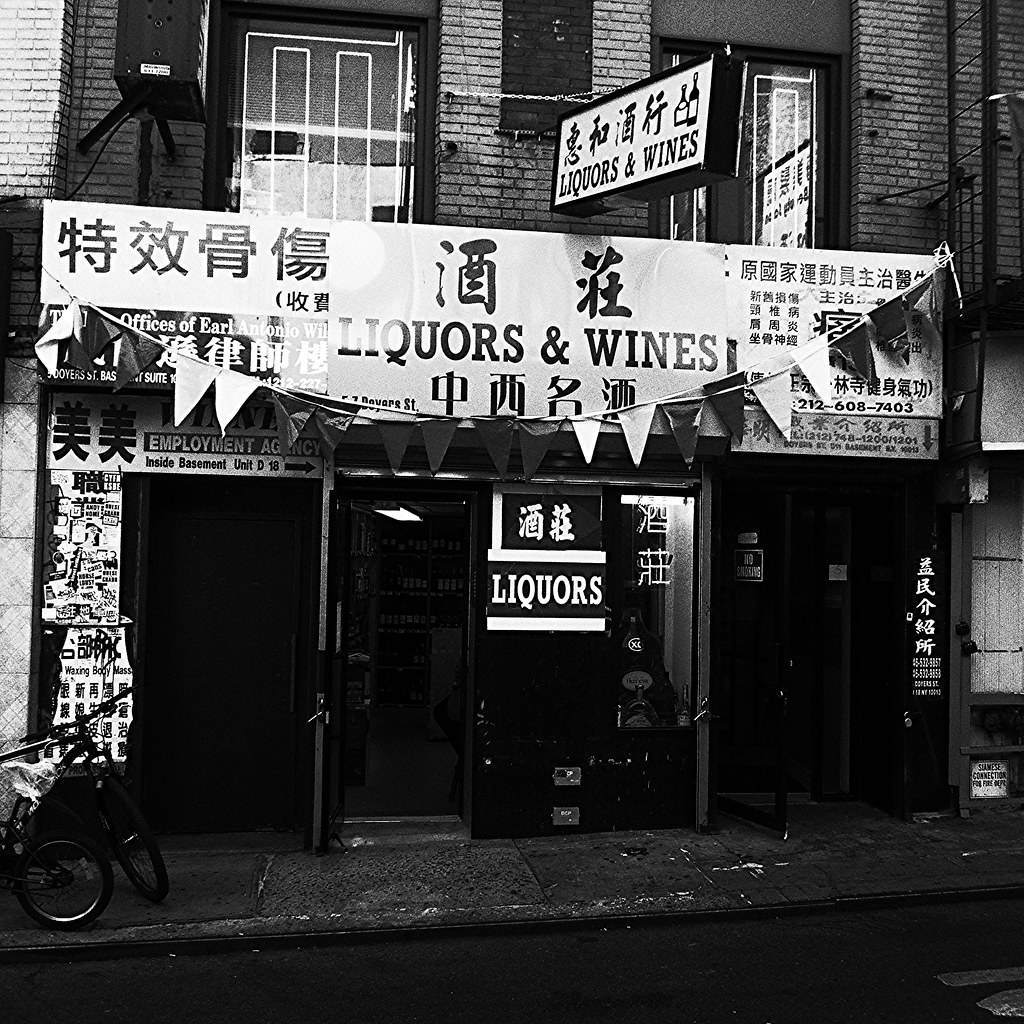This black-and-white photograph captures the gritty facade of a liquor store located in what appears to be Chinatown. The scene is dominated by an old, two-story brick building with a slightly dingy and weathered appearance. The storefront's first floor features multiple entrances: a swinging door on the left side that reveals a lit interior, and another door on the right marked with a partially obscured "No Smoking" sign. Between these doors is a wall bearing a large, worn sign that boldly announces "LIQUORS" in English, flanked by Chinese characters both above and below.

A prominent white vertical sign runs down the middle of the building, prominently featuring "Liquors and Wines" in bold black print, surrounded once again by Chinese script, and an additional segment advertising the offices of Earl Antonio alongside a phone number indicative of a New York location. Numerous ragged, weathered handbills with Chinese text are plastered on the far left wall, contributing to the building’s sense of age and urban decay.

Above, the second story is adorned with a window shrouded in what appears to be a combination of window shades and paper coverings. To the right, another window reflects the street view, while a fire escape clings to the building's facade.

Additional signage includes a smaller sign jutting out from the building, also proclaiming "Liquors and Wines," embellished with a graphic of a wine bottle and more Chinese characters. A string of triangular flag banners stretches across the scene, and the sidewalk below is dark and grungy. A bicycle is parked in front of the store, completing the urban landscape.

Overall, the photograph evokes a sense of gritty realism, highlighting the cultural blend and worn aesthetic of a Chinatown liquor store amid a black-and-white street setting.